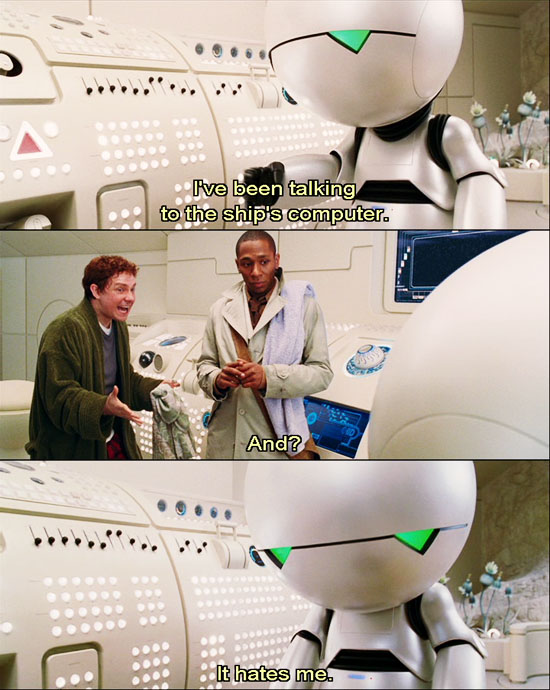In this meme, which appears to be a scene from the movie "Hitchhiker's Guide to the Galaxy" and formatted in three stacked rectangles, we follow the narrative of a white, round-headed robot interacting with the ship's computer. 

In the top frame, the robot, characterized by its large head and green triangular eyes, walks past intricate computer panels adorned with white lights, black knobs, and buttons. The overlaying text reads, "I've been talking to the ship's computer." 

The middle frame features two characters: one is a black man wearing a tan trench coat with a brown bag slung over his shoulder and a purple towel, and the other is a red-haired man dressed in a green robe and gray shirt. This scene captures the red-haired man with an open mouth and gesturing hands while the other man stands beside him, both looking at the robot. The text in this panel merely says, "and."

In the bottom frame, there's a close-up of the robot's face, clearly showing its two eyes and a noticeably downcast expression. The caption for this frame reveals the robot's dismay: "it hates me." The overall caption of the meme, therefore, reads: "I've been talking to the ship's computer, and it hates me," highlighting the humorous, yet sad, plight of the depressed robot.